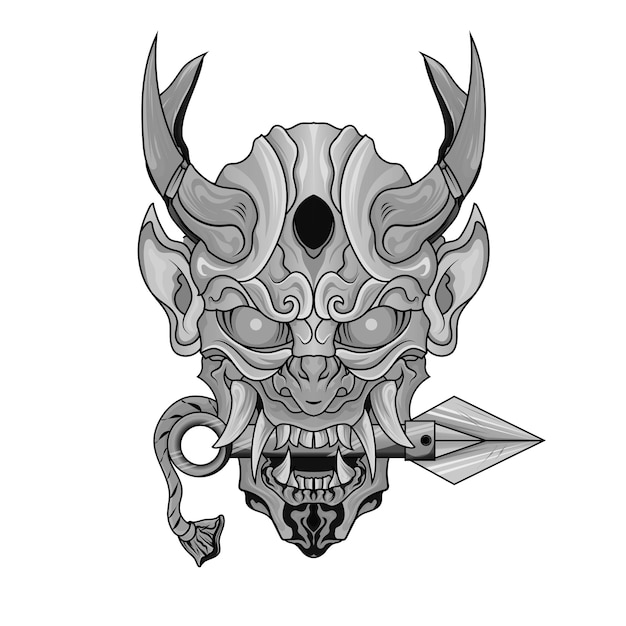The image is a computer-generated artwork, created in portrait orientation, resembling a demon's head with an intricate, gray-toned design against a plain white background. The demon's face is oval, with a sharp, pointed chin, and features prominent, elaborate, dark gray horns curving upward from each side of its head. The skin appears wrinkly, giving the face a textured appearance. At the center of the forehead, between the horns, there is a distinct black oval.

Two pointed ears jut out from each side of the head, and the eyes are a piercing light gray with even lighter dots in the centers, lending the creature an intense gaze. The mouth is slightly open, revealing long, pointed fangs. Clenched between its teeth is a horizontal dagger with a sharp triangular blade on the right end and possibly a rope hanging down from the left. The dagger resembles a shinobi knife, adding to the menacing look of the creature. The chin of the demon head sports a small, goatee-like detail, enhancing the overall sinister and detailed appearance of the artwork.